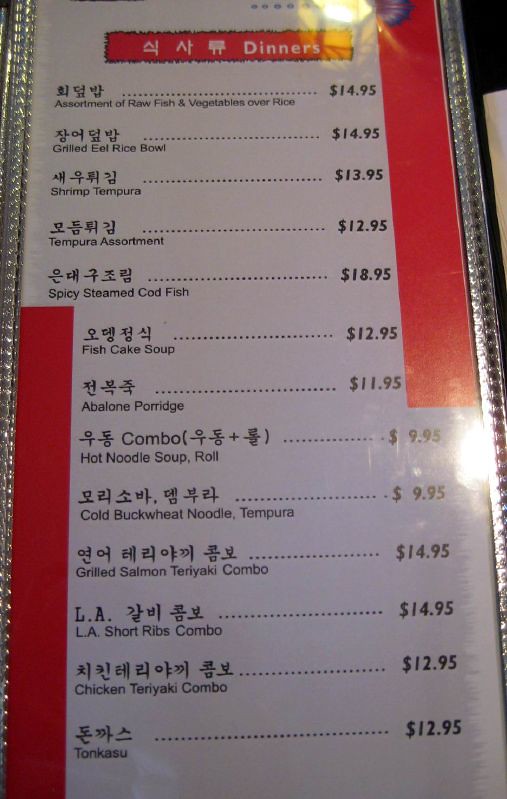The image showcases a neatly framed menu, encased in a sleek metal frame with a glass front, suggesting it is mounted on a wall. The focus of the photograph zooms closely on the menu itself, omitting other surroundings. At the top of the menu are the words "Dinners" accompanied by Korean characters.

The menu items are listed in two languages: Korean on the left side, with the corresponding English translations and prices in dollars to the right. The white paper backdrop of the menu is accentuated by two decorative red bars: one extends from the top right corner down slightly past the midpoint, and the other from the bottom left corner up similarly past the midpoint.

Here is a detailed list of the menu items:

1. Assortment of raw fish and vegetables over rice
2. Grilled eel rice bowl
3. Shrimp tempura
4. Tempura assortment
5. Spicy steamed codfish
6. Fish cake soup
7. Abalone porridge
8. Hot noodle soup roll
9. Cold buckwheat noodle
10. Grilled salmon teriyaki combo
11. LA short ribs combo
12. Chicken teriyaki combo
13. Tonkatsu

Above these items, there is additional Korean writing mentioning "combo" with further details in parentheses. Although many dishes have Japanese names, the script and distinctive circles in the characters confirm the language as Korean.

This detailed depiction highlights the multicultural culinary offerings, emphasizing the authentic Korean writing style contrasted against a backdrop of Japanese cuisine terminology.